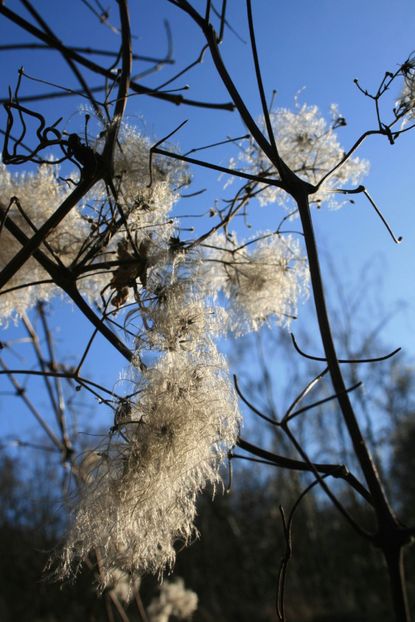The photograph captures a close-up of tree branches adorned with delicate, cotton-like flowers positioned against a light blue, cloudless sky. The image is rectangular, twice as wide as it is tall, with the lightest part of the sky on the right side, hinting at the direction of the sunlight. The primary branch emerges from the bottom right corner and extends upward, splitting into a 'V' formation one-fourth of the way up. The left branch, slightly thinner, extends toward the left and center of the image, showcasing numerous smaller branches peppered with wispy, feather-like flowers. These flowers, consisting of small brown bulbs and light gray strands, evoke a sense of airy fragility and resemble cotton balls. The right branch is thicker but sparsely decorated with these white fibrous blooms. Surrounding the foreground branches, taller, leafless trees form a blurred, skeletal backdrop, enhancing the scene’s natural and serene outdoor setting. The dead-end stems without flowers add a stark contrast, emphasizing the prominence of the blooming cotton-like flowers.